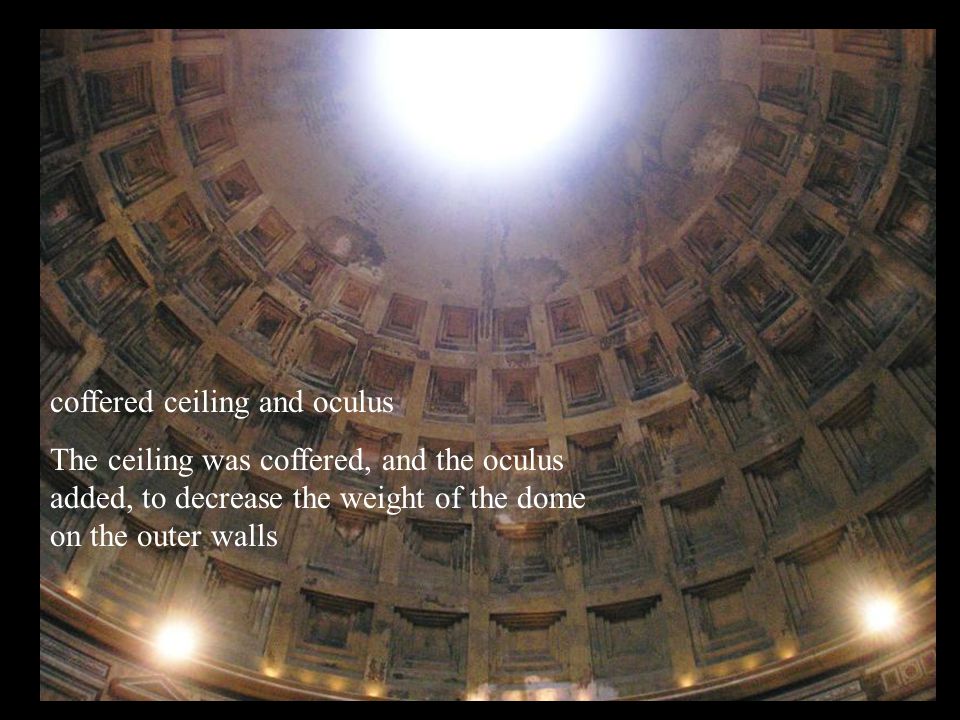The image captures the interior of a grand, well-architected building, focusing on an ornate ceiling with a domed structure. The top center of the dome features a bright, natural white light shining through an oculus, illuminating the intricate details below. The ceiling displays a coffered design, characterized by a grid pattern of indented squares that form a geometric pattern and reduce the dome's weight on the outer walls. Surrounding the edge of the dome are several artificial lights, with four smaller lights evenly spaced and two brighter lights positioned on the right and left sides of the image. The photograph includes a black border framing the composition, and white text located on the left side of the image reads: "Coffered ceiling and oculus. The ceiling was coffered and the oculus added to decrease the weight of the dome on the outer walls." The scene is predominantly colored in shades of black, brown, white, gray, tan, and yellow, emphasizing the architectural craftsmanship and the ambient light effects within the indoor setting.